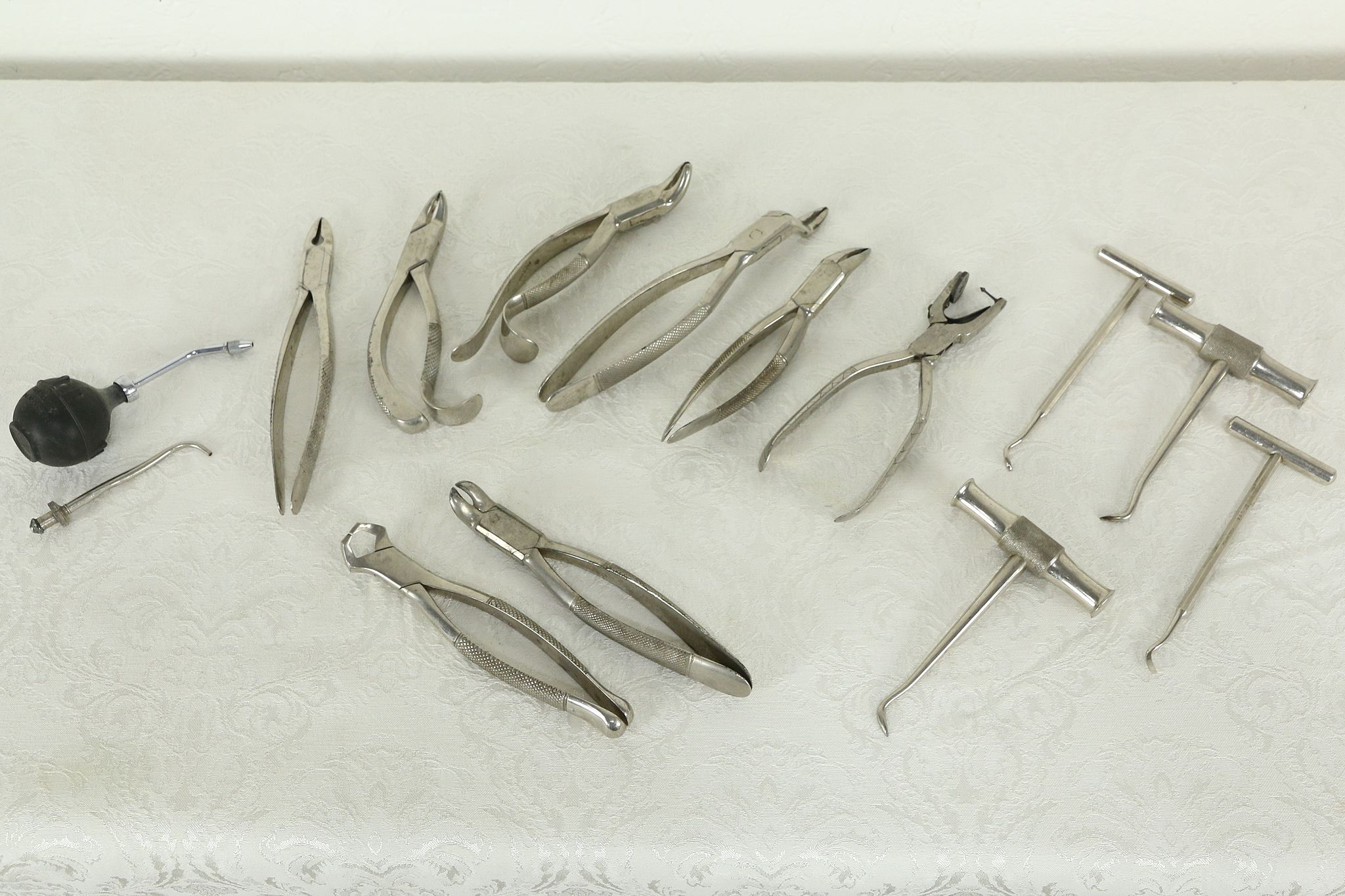This detailed photograph captures an array of dental instruments meticulously arranged on a white, embroidered tablecloth. A total of 14 silver, metal tools are displayed. On the far left, there is a distinctive tool featuring a black bulb on one end and a silver metal component. Directly beneath it, another metal instrument can be seen. To the right of these are six different types of plier-like dental tools, each varying slightly in shape and size. In the center, the arrangement continues with two additional long, plier-like instruments. The rightmost section showcases four more instruments that resemble tiny hammers. These hammer-like tools are small, approximately two to three inches in length, with thin, needle-like metal parts and small hammer heads at the top. The entire setup is placed against a white backdrop, and the intricate embroidery of the tablecloth adds a refined touch to the clinical precision of the dental instruments.